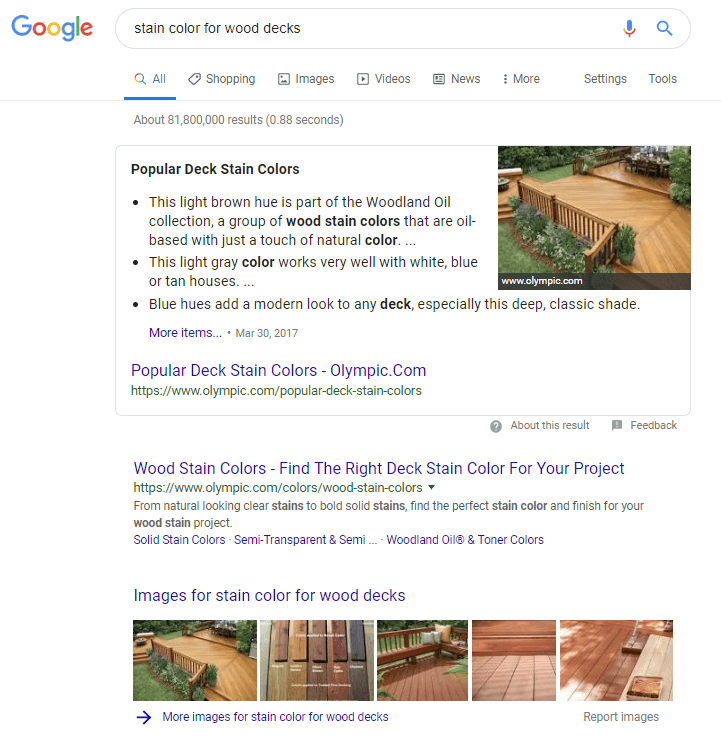The image depicts a Google search results page with the query "staining colors for wood decks" entered into the search bar. At the top of the page, the typical Google tabs—All, Shopping, Images, Videos, News, More, Settings, and Tools—are present, with the "All" tab highlighted in blue and a blue line running underneath it. The search query yielded approximately 81,800,000 results in 0.88 seconds.

Highlighted search results include a description of popular deck staining colors, emphasizing a light brown hue from the Woodlands Oil Collection. This collection features oil-based stains with subtle natural colors. Another featured color is a light gray, mentioned for its compatibility with white, blue, and tan houses, creating a modern look when paired with deep blue hues.

A photograph of a deck displaying a golden brown color is shown, accompanied by the text "www.olympic.com." Below the image, a link titled "More items" dated March 30, 2017, directs to more information about popular deck staining colors on olympic.com.

Additional search results focus on wood staining options, presenting various Olympic brand products. These include clear stains for a natural look and bold solid stains for more pronounced color. The page also mentions semi-transparent and translucent stain options, highlighting the variety of finishes available for different wood staining projects. There are links to further details and feedback options, inviting users to explore and select the perfect stain for their needs.